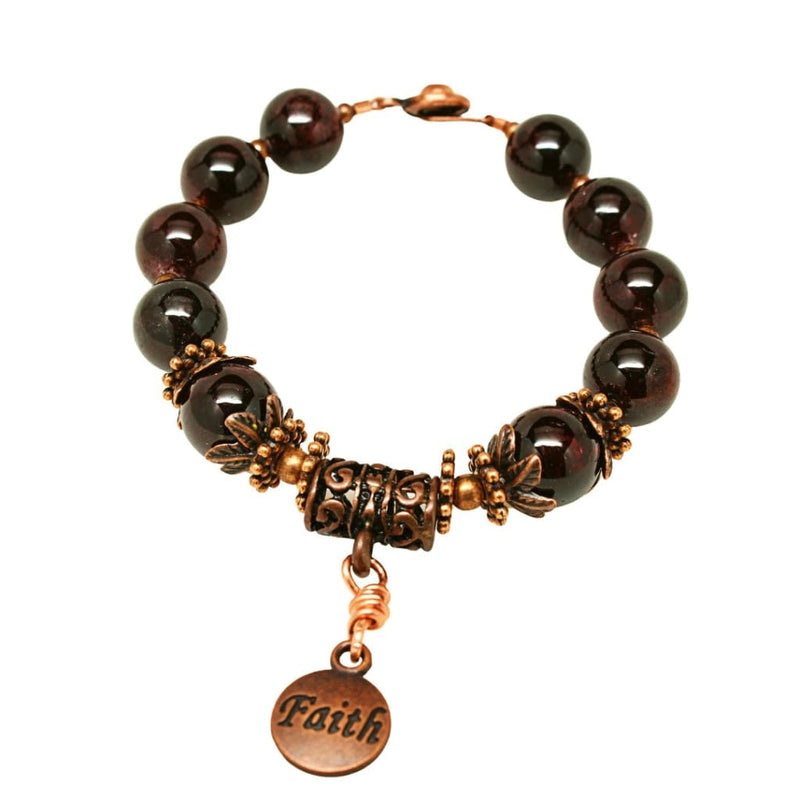This detailed close-up image captures a sophisticated beaded bracelet adorned with dark, almost black spherical beads that might be obsidian or onyx, exhibiting a glossy, glassy finish. Interspersed among these shiny beads are small, intricate metal pieces with a leaf or plant-like appearance, displaying a dark brass or copper hue. The centerpiece of the bracelet features a cylindrical form from which a circular metal piece extends, connecting to a wire-wrapped copper charm. This charming pendant bears the word "Faith" engraved in black. The bracelet's clasp is slightly out of focus in the background, hinting at its function to secure the bracelet around the wrist. The photograph's white background accentuates the delicate details and the blend of dark beads with metallic elements.